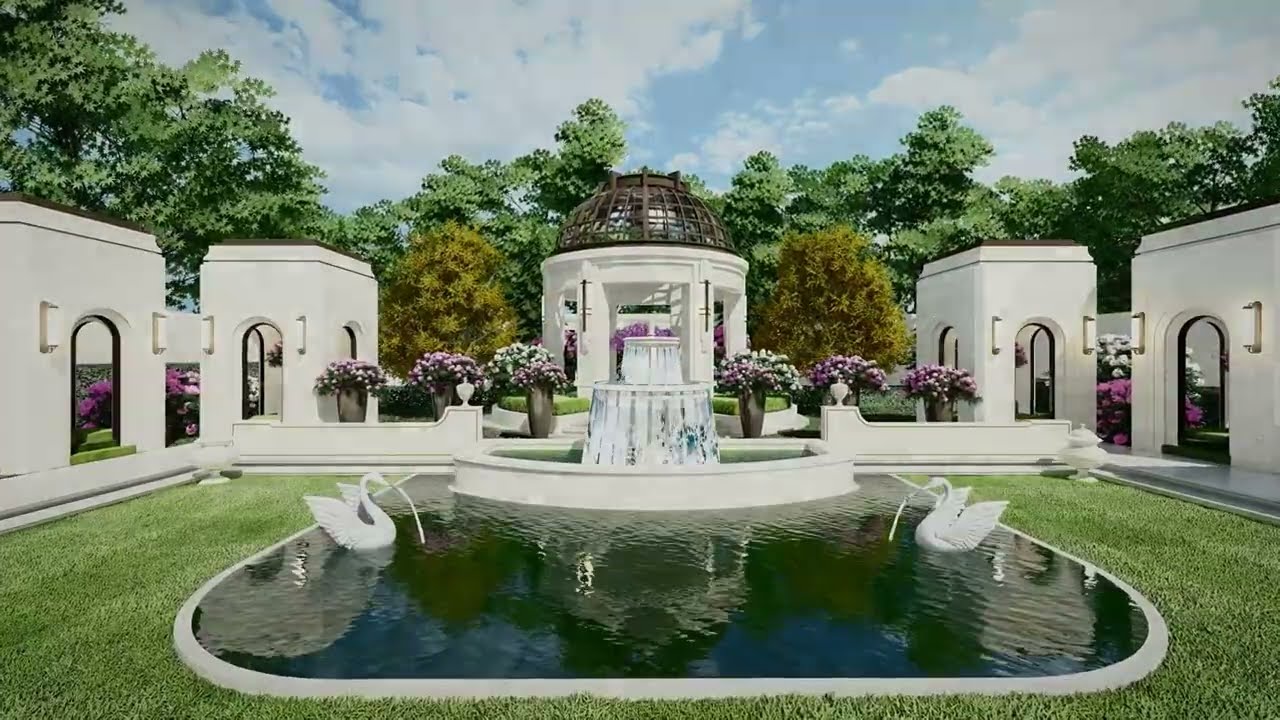In this opulent garden scene, a central dark blue reflecting pool features an ornate fountain composed of three tiers, softly cascading water. On either side of the pool, elegant white swan statues spout arcs of water from their beaks. The pool is bordered by a pristine white curb and is ensconced in a meticulously manicured green lawn. Flanking the fountain are tall, white vases adorned with purple, white, and pink flowers, positioned symmetrically—three on each side.

In the background, a charming gazebo with a dome roof, supported by white pillars, hosts an array of white flowers within. Adjacent to the gazebo are square tower-like structures, two on each side, giving an appearance of arched entrances that could provide shade. The scene is framed by a row of green and yellow-tinged trees under a bright blue sky with scattered white clouds, creating a lush and serene atmosphere.